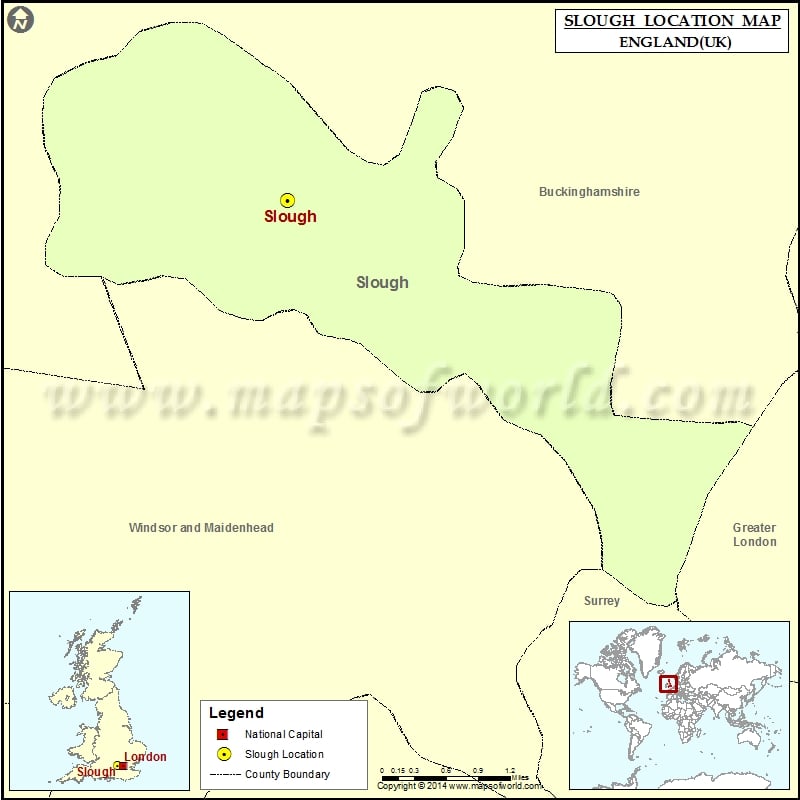This detailed map depicts the region of Slough within the UK. In the top right corner, a white box reads "Slough Location Map, England, UK." The primary map, which occupies the majority of the space, includes a yellow background with several areas labeled in gray text, such as Buckinghamshire near the top, Windsor and Maidenhead near the bottom left, and Greater London and Surrey. The area of Slough is highlighted in light mint green and is marked in red text, with additional gray text labels for "Slough."

A smaller inset map of the UK is located in the bottom left corner, showing the national capital, London, in a red square. This inset helps to contextualize Slough's position within the broader country. Next to this inset, the legend explains the map's color codes: red signifies the national capital, yellow indicates the Slough location, and black denotes county boundaries. Slough's location is specifically marked by a yellow circle with a bullet inside.

Additionally, the bottom right corner features a world map, pinpointing the specific region discussed. The entire image is overlaid with the source website's address, "www.mapsofworld.com." This map, with its varied colors including gray, yellow, black, white, light blue, and red, serves as an informative tool, possibly intended for educational purposes, to understand Slough's geographic and administrative context within the UK.